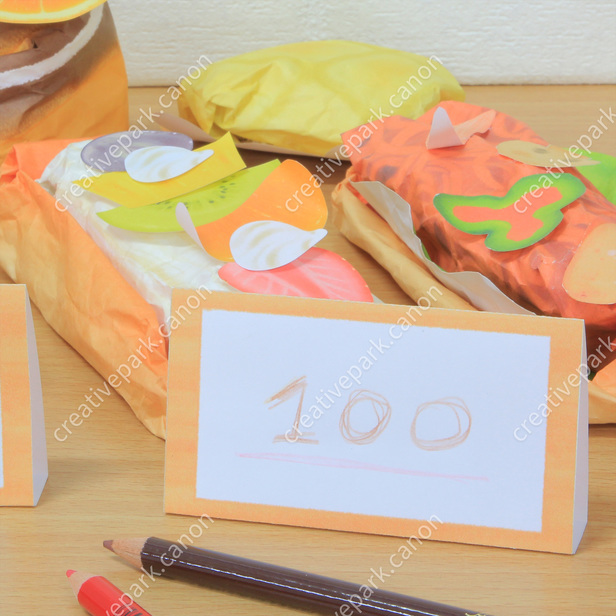This photograph, possibly an advertisement, is marked with a diagonal watermark reading "creativepark.canon". It showcases a brown table adorned with various arts and crafts items. At the forefront of the image lie a brown and a red pencil, as well as a rectangular piece of paper standing vertically, bordered in orange, and featuring the number "100" penciled in brown with a red underline. Surrounding this centerpiece is an assortment of creatively packaged items, resembling sandwiches wrapped in different colors of paper such as yellow and orange. Adorned with cut-out paper vegetables like bell peppers, onions, and garlic, these packages convey a whimsical, handmade aesthetic.